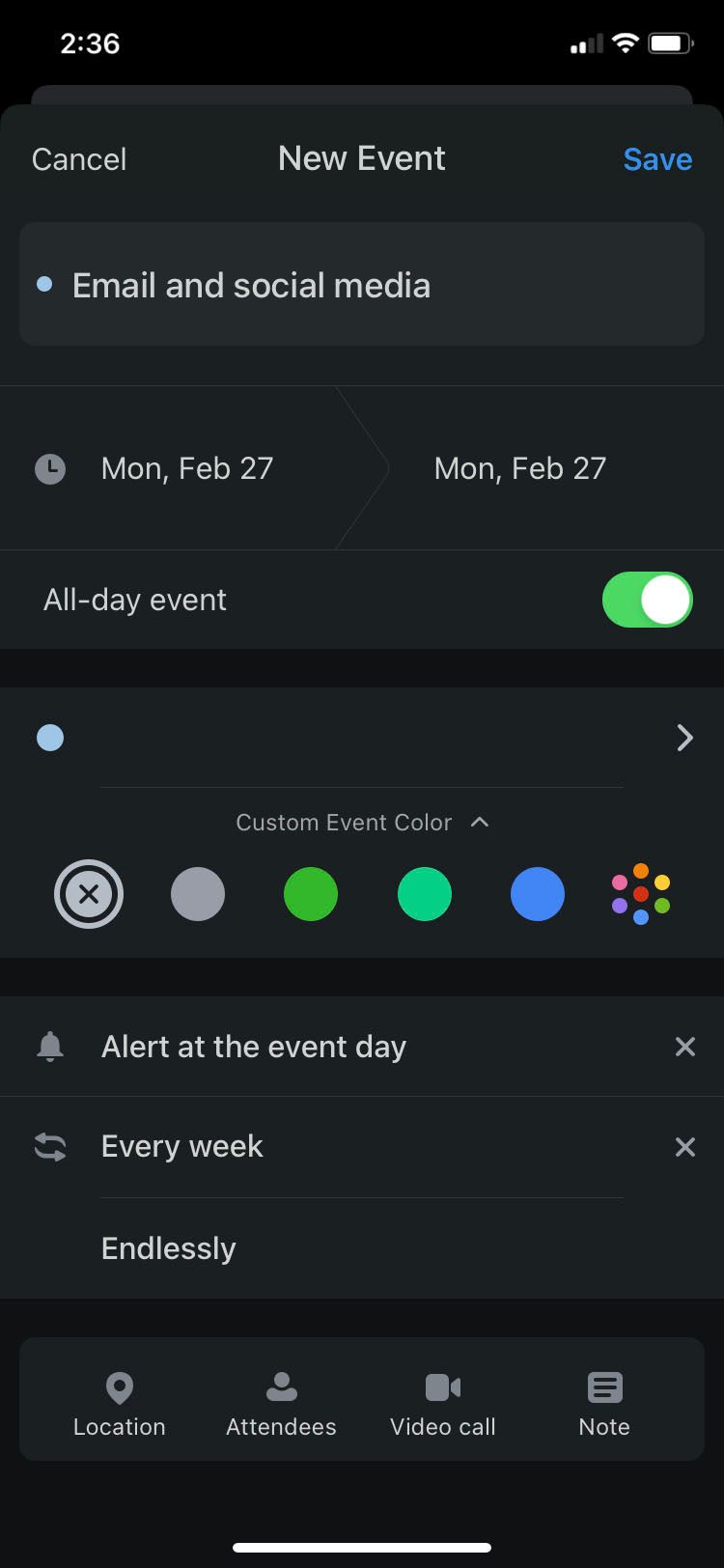This screenshot of an iPhone display captures a detailed view of the Calendar app interface used for event scheduling. In the top left corner, the current time is shown as 2:36. On the top right, the network signal is visible. The interface includes navigation options such as "Cancel," "New Event," and "Save" at the top. The screenshot specifically indicates an event labeled "Email and Social Media" scheduled for Monday, February 27, marked as an all-day event and set to repeat every week. Additional event details are visible, including the location, attendees, options for a video call, and notes. The structured layout and options suggest a focus on organizing and managing calendar events efficiently.